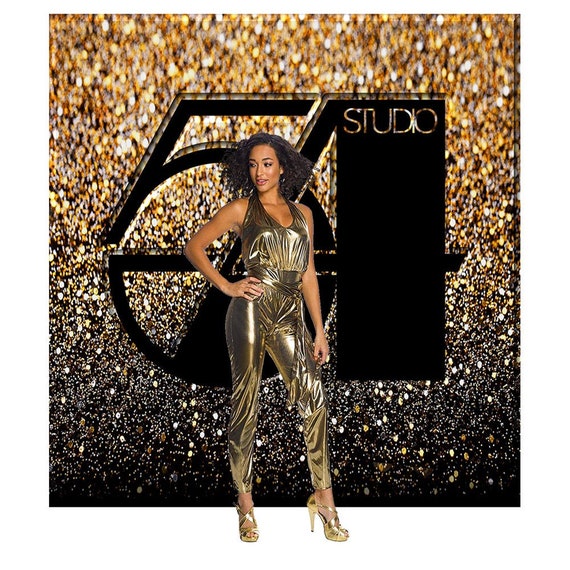This advertisement for Studio 54 is a dazzling display of 70s disco revival, featuring an African-American woman adorned in a shimmering gold lamé jumpsuit complemented by matching gold lamé peep-toe heels. Her frizzy, curly black hair frames her face, as she confidently stands with her right hand akimbo, gazing off to the side. The background is a radiant, shimmery cascade of gold glitter at the top, which gradually fades to a darker, silvery-black hue at the bottom, enhancing the opulent atmosphere. Dominating the backdrop is a large, stylish logo of the number "54" in black, with "Studio" emblazoned in gold lettering within the top part of the "4". The overall image focuses on the contrast of gold, black, and brown tones, encapsulating the glam and glitz of the iconic Studio 54 era.